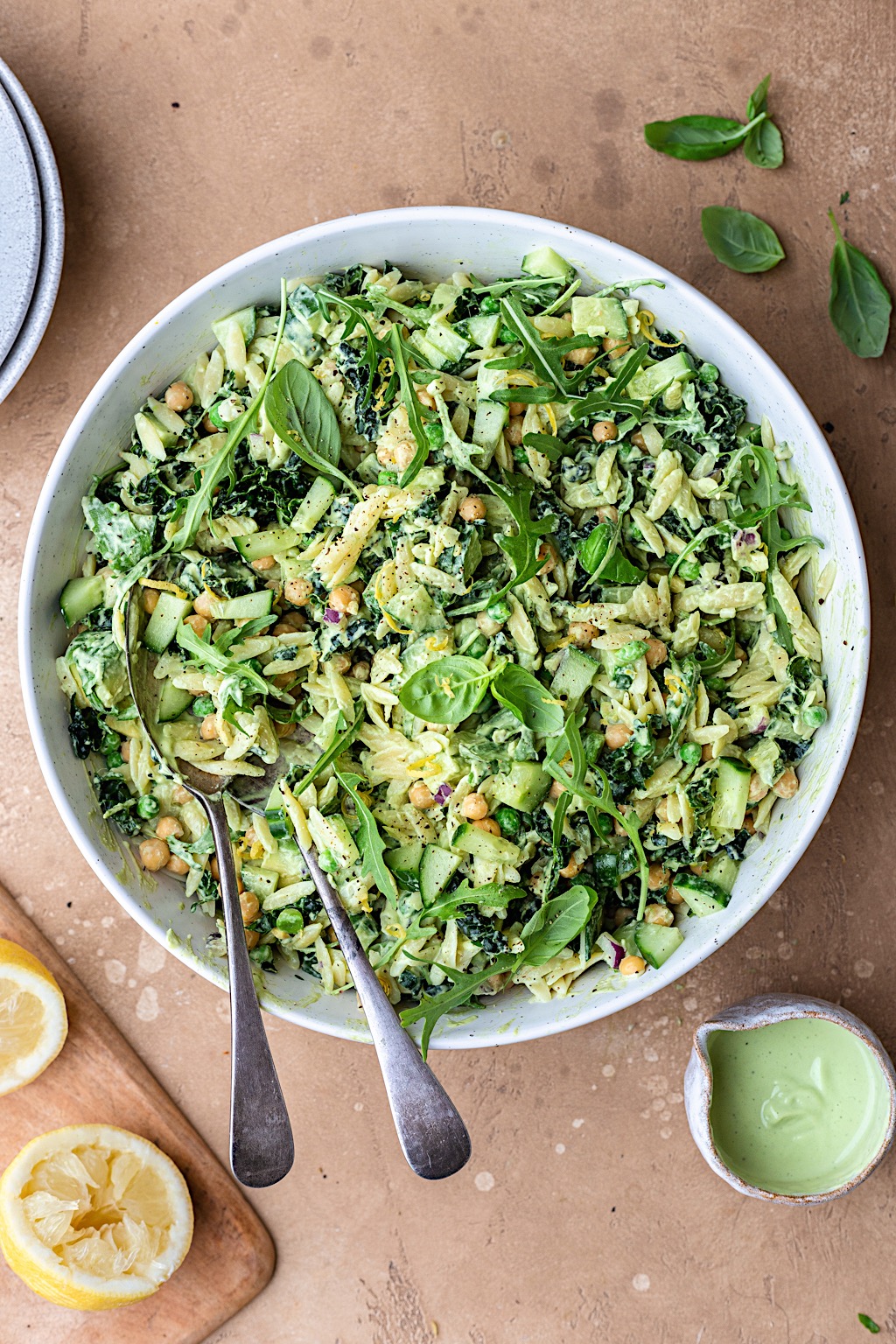This vibrant top-down photograph captures an artfully arranged chopped salad in a large white bowl, set on an unfinished wood table. Dominated by rich greens, the dish features a mix of fresh spinach leaves, basil, and lettuce, interspersed with creamy orzo pasta, chickpeas, and slices of bright red onions. Nestled alongside these ingredients are small, uncut leaves which accentuate the freshness of the salad. Two silver spoons are placed, one on top of the other, to the side, ready for serving. 

Adjacent to the bowl on the bottom right, a small container with a spout holds a bright green dressing that blends seamlessly into the salad, adding a subtle creamy texture without overpowering the colors. To the left of the dressing, on a wooden cutting board, lies a halved lemon, its squeezed state suggesting it was freshly used to add a zesty kick to the dressing or the salad itself. The scene is complemented by aesthetically arranged spinach leaves on the table edges and a partially visible stack of plates, enhancing the rustic yet refined food photography composition.